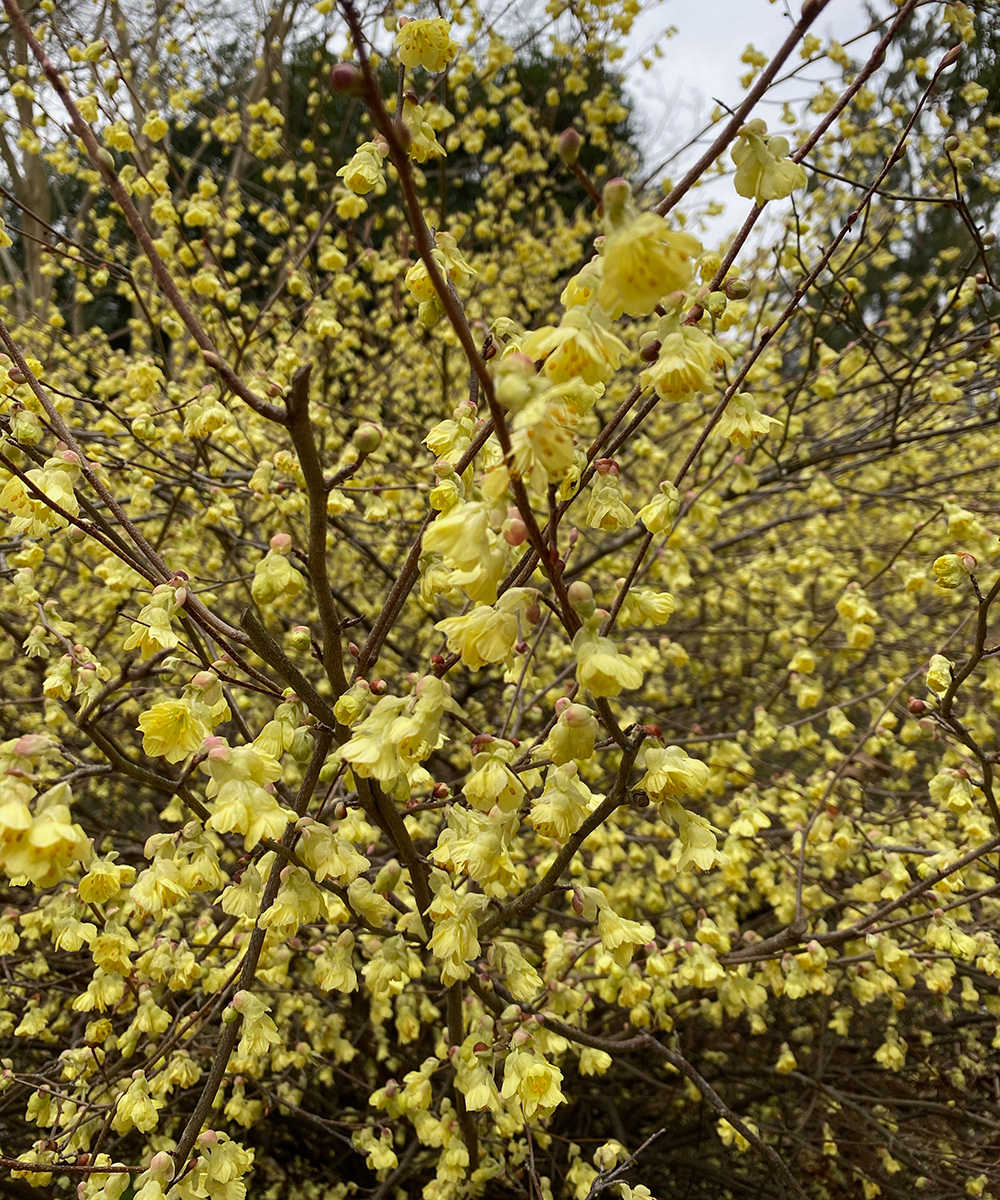A close-up photograph captures the vibrant detail of a Scotch Broom plant. The thin, brown branches are adorned with clusters of small, vivid yellow flowers. This tight focus highlights the intricate structure and color of the plant, drawing attention primarily to the center of the bush. In the background, blurred green foliage fades into a backdrop of light blue sky, adding depth to the image. To the left, about a foot and a half into the background, dense greenery contrasts with a small visible patch of sky, while on the right, another section of bush remains softly out of focus, ensuring the Scotch Broom takes center stage in this botanical portrait.